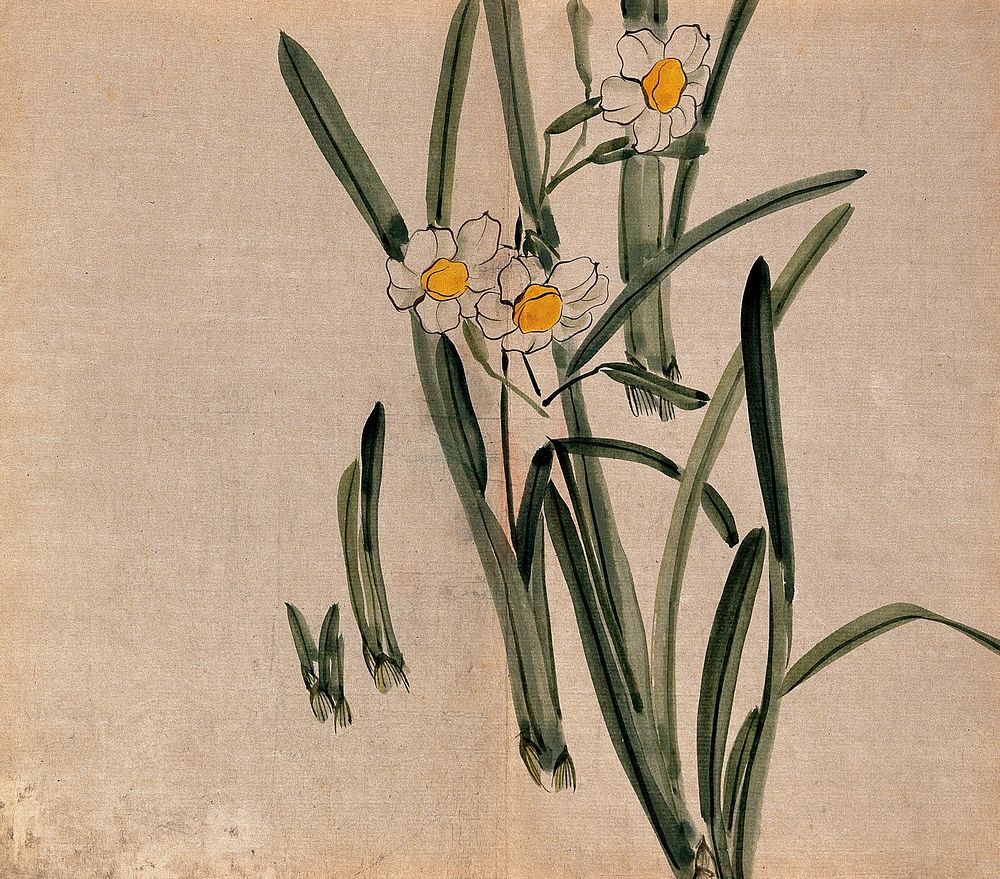The image depicts a watercolor painting on a tan, aged canvas, possibly resembling worn parchment. The canvas displays darker, weathered patches in the bottom left, adding to the rustic charm. The focal point of the painting is a selection of small white flowers with yellow centers, likely daffodils, grouped slightly to the right of the canvas center. These blooms are accompanied by dark green stems, which exhibit a mixture of broad, straight, and slightly listing growth patterns. The leaves are mostly symmetrical and extend both vertically and horizontally in long, light green and dark green hues. Notably, there are two prominent flowers with white petals and yellow centers clustered near the middle of the image, while a similar bloom emerges from another stem positioned towards the top right, facing right. Additionally, a few unattached stems, devoid of flowers, stretch out toward the left center of the canvas, adding depth and complexity to the botanical arrangement. The watercolor technique delivers a soft, smudgy effect, enhancing the overall delicate and aged appearance of the piece.